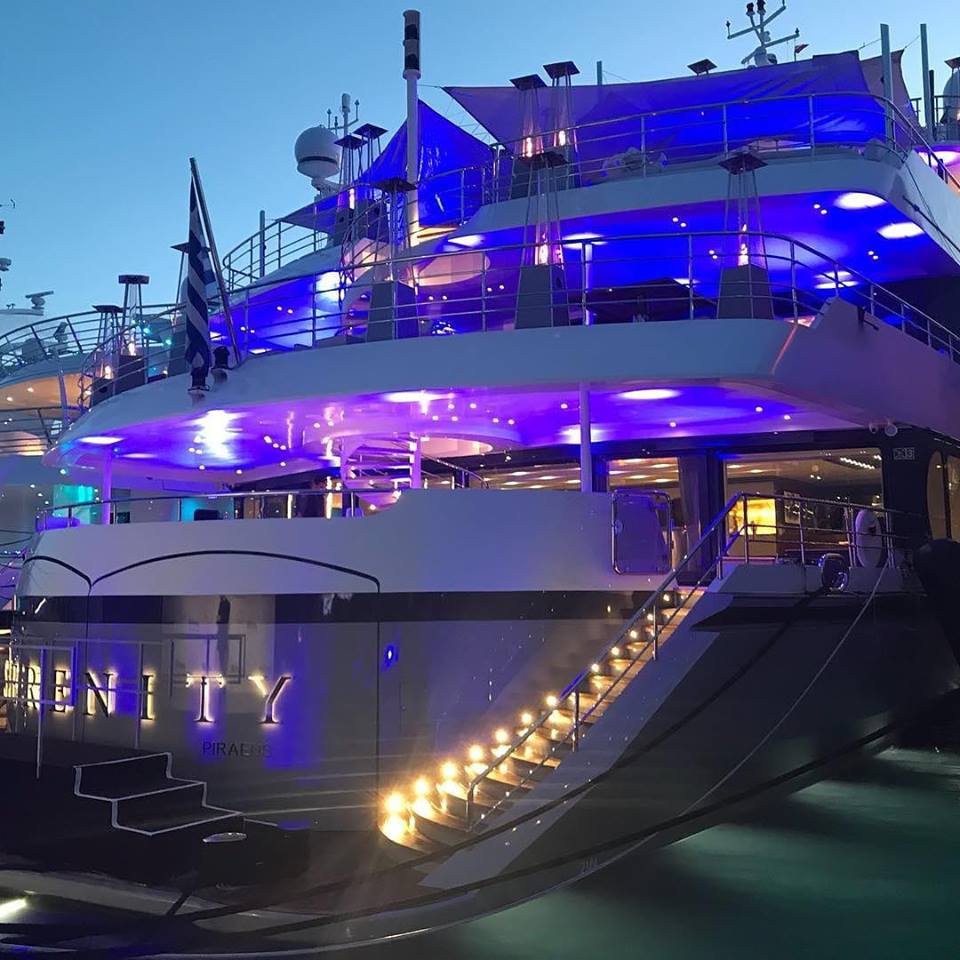The image depicts a large structure resembling a cruise ship, though it appears to be on land rather than in water, possibly a building designed to look like a ship. The photograph is taken during dusk or dawn, with various lights accentuating its features. There are three or four stories to the structure, each outlined with purple and blue lighting. 

In the foreground, a well-lit staircase with individual lights on each step ascends to the first level, which is bathed in yellow light. The name "Serenity" is partially visible in yellow letters on the left side of the image. Above the first level, the second level features a flagpole with an American flag, though the details of the flag are not entirely clear due to the lighting and time of day. The second and third levels also have railings, and additional blue lighting appears on the ceilings of these floors. 

In the upper left corner of the image, a sliver of blue sky is visible, hinting at the outdoor setting. The image also shows hints of boat masts and sails, suggesting the structure might be docked at a marina.